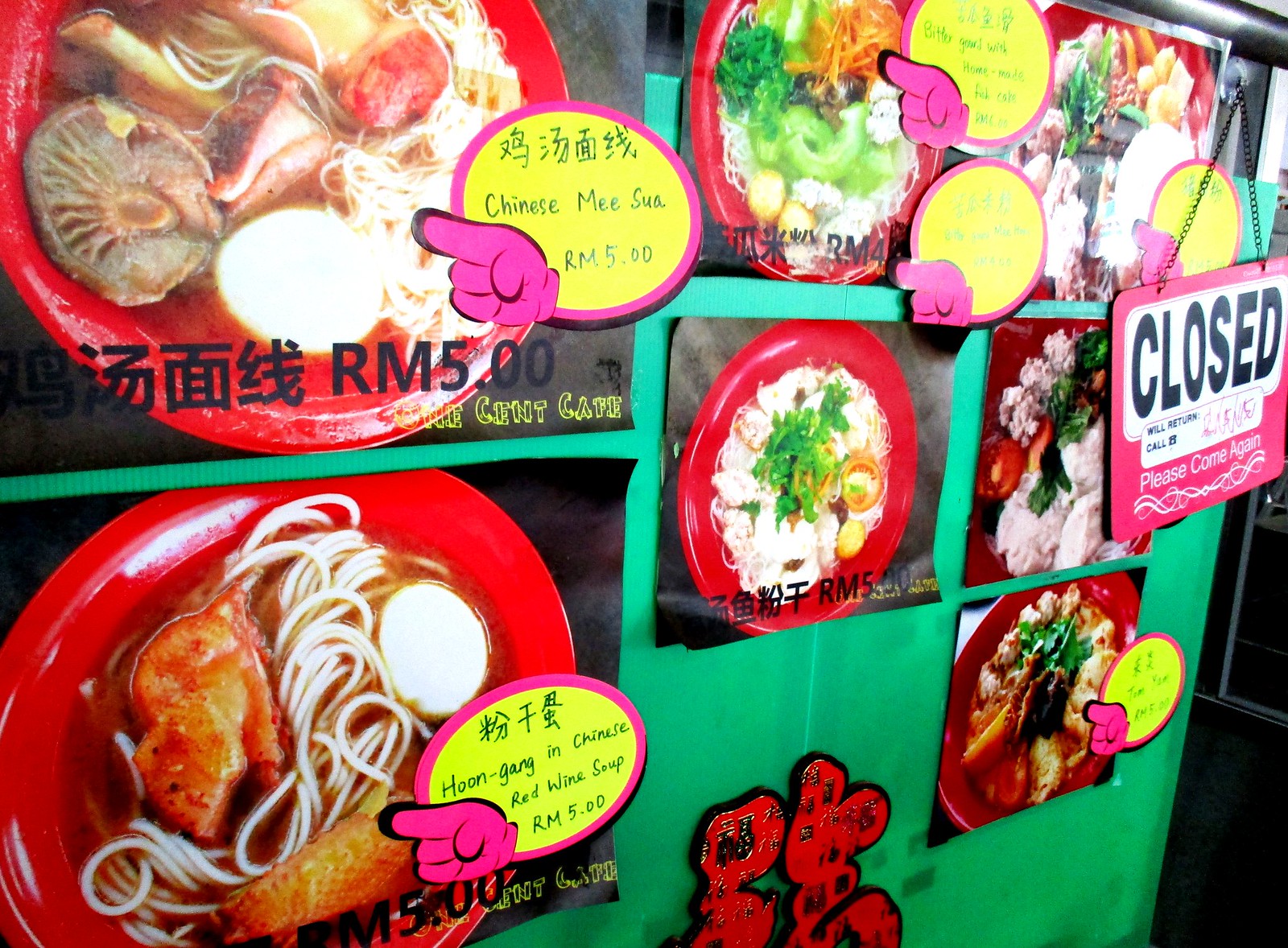The photograph showcases a Chinese restaurant menu displayed on a green wall. The menu features various dishes with corresponding prices in RM, such as RM5. The images of these dishes are centrally located against a black background. Each dish includes a circular label with an arrow pointing towards it, highlighting the name and price. Clearly visible are the dishes "Chinese Mei Sua" and "Hong Kong in Chinese Red Wine Soup," indicated by depictions of food in red bowls with labels marked by colorful borders. A prominent "Closed" sign hangs on the right side, featuring text on a red background that reads, "Closed, Please Come Again," with a contact return notice. Red plates with food are also visible, enhancing the presentation of the meal options.